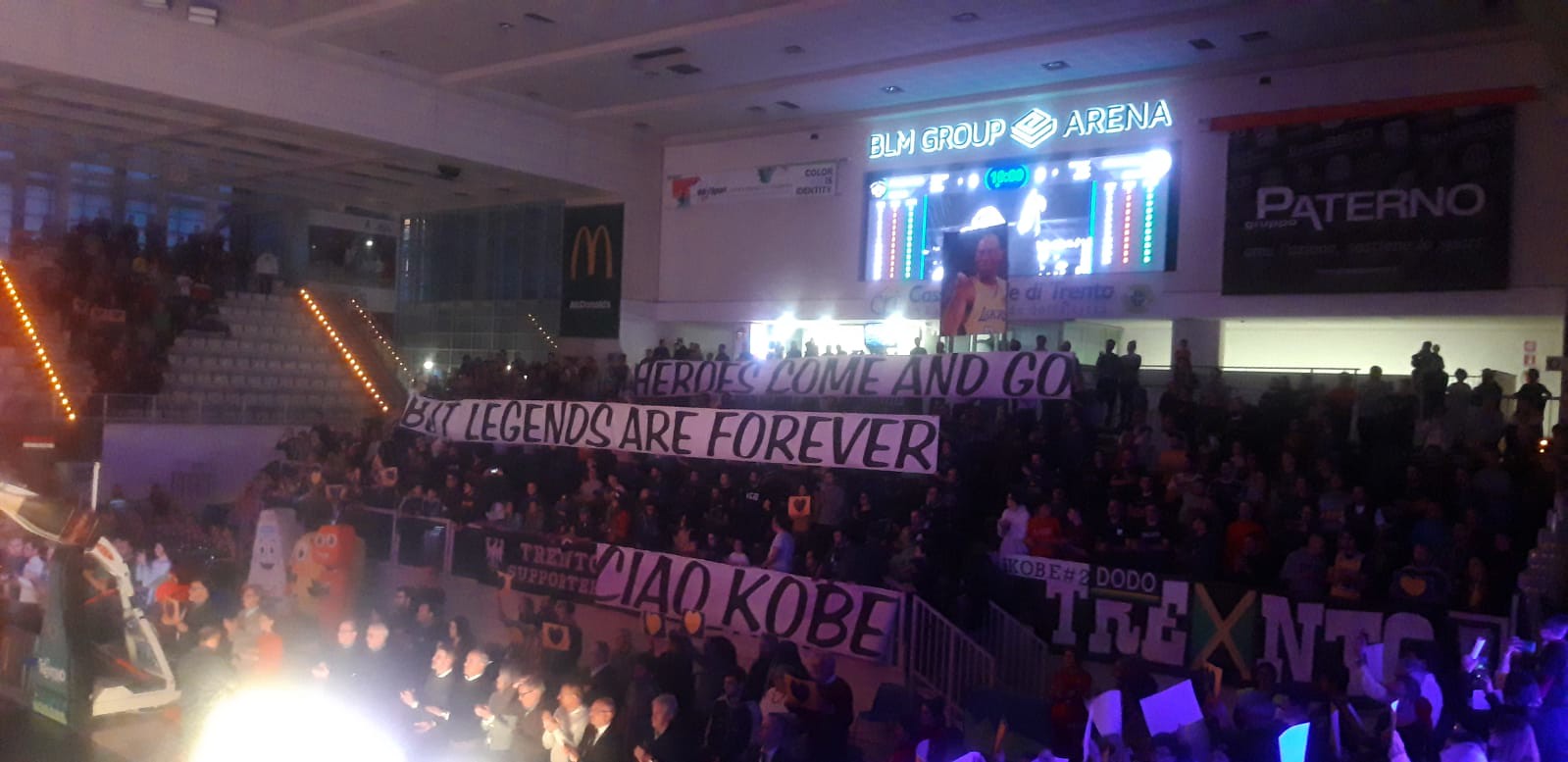The image depicts a large indoor stadium filled with a substantial crowd positioned primarily at the bottom center. Above the crowd, there is a prominent digital screen displaying "Beyond BLM Group Arena," with additional signage below it. One of these signs reads, "Heroes come and go, but legends are forever," possibly in remembrance of an influential player such as Kobe Bryant. The arena's upper left section features empty seats, and another screen with the word "Paterno" appears to the right of the central screen. The setting gives the impression of an evening event, illuminated by a bright white light situated near the lower left of the image. The scene is a vivid mix of colors including white, yellow, orange, blue, purple, green, tan, and black, contributing to the dynamic ambiance of the arena. Banners and signs held by attendees enhance the emotional and commemorative atmosphere of the gathering.